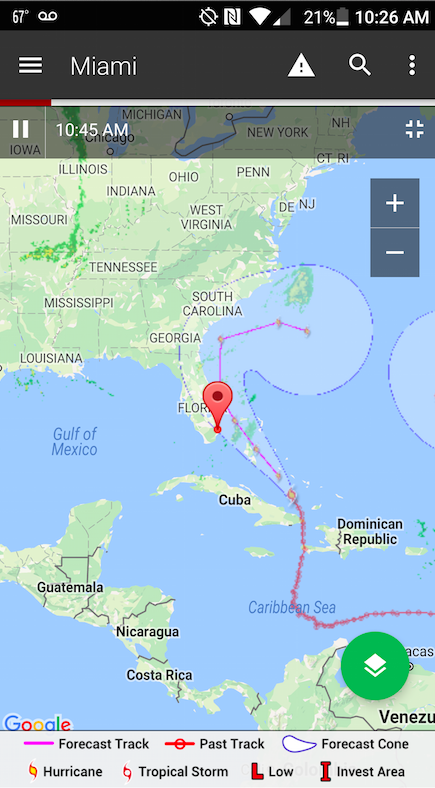This is a screenshot from a weather application on a smartphone. At the top of the screen, there is a black rectangle displaying several indicators. On the top left, it shows a temperature of 67 degrees accompanied by an icon of upside-down glasses. Moving right, there is a cross-line through an option, a sideways Z, a full Wi-Fi signal bar, and a cellular reception with one or two bars out of four. Following these, the battery icon shows 21% and the current time is 10:26 a.m.

Below this, there's a larger gray rectangle with three horizontal lines and the word "Miami" in white text. To its right, there are icons for a notification (a stop exclamation mark), a search function, and three vertical dots, typically representing a menu.

The main portion of the screenshot is a map featuring parts of the United States, including Florida, as well as Cuba, Venezuela, and Guatemala. Over Florida, there's a red check mark indicating a significant point. A forecast track, represented by a purple line, shows a storm originating southeast of Florida and moving north past the southeastern tip of Florida, continuing through Georgia and South Carolina, and eventually heading into the Atlantic Ocean. This path is highlighted with a blue outline, denoting a forecast cone, which is filled with a light blue area.

At the bottom of the picture, a legend explains the map's indicators: a purple line for the forecast track, a red line for the past track, and a blue outline with light blue inside for the forecast cone. On the bottom right, there is a green circle with two white squares inside.

Overall, the image provides a comprehensive look at the forecasted storm’s path and relevant weather information for the region.